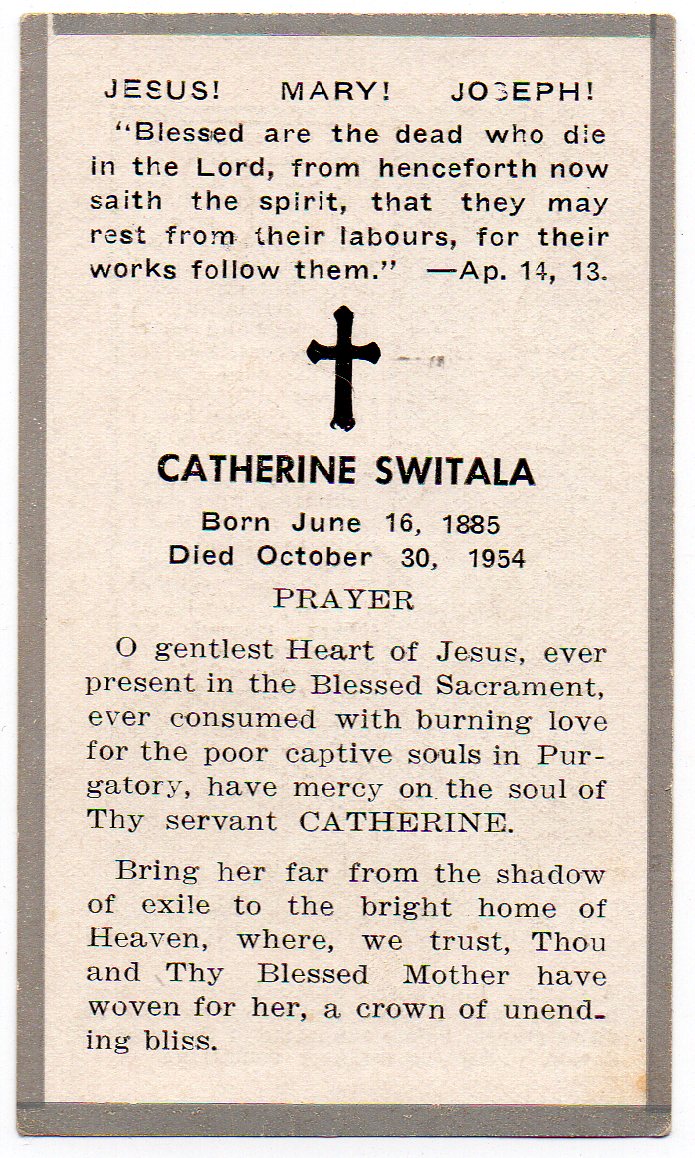The image shows an aged prayer card with a light gray background bordered by a darker gray edge. Centered at the top in emphatic lettering are the words "Jesus! Mary! Joseph!" followed by a scripture quotation: "Blessed are the dead who die in the Lord, for henceforth, now, saith the Spirit, that they may rest from their labors, for their works follow them." Below this, prominently displayed, is the name "Katherine Switala" with a black cross above it. The card details that Katherine Switala was born on June 16, 1885, and passed away on October 30, 1954. Beneath her name, a prayer implores, “O Gentle Hearts of Jesus, ever present in the blessed sacrament, ever consumed with burning love for the poor captive souls in purgatory. Have mercy on the soul of thy servant, Katherine. Bring her far from the shadow of exile to the bright home of heaven, where we trust, thou and thy blessed mother hath woven for her a crown of unending bliss.” The text is printed in black on the paper, which, due to its age, appears somewhat dirty.